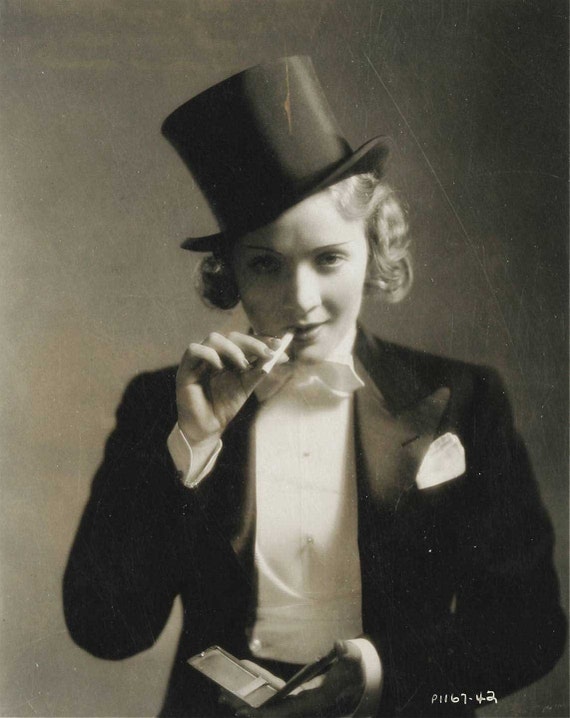This striking black-and-white photograph features a light-skinned woman with short, curly blonde hair that falls to her ears, giving her a distinctive, vintage look. She dons a classic black tuxedo complete with a white shirt, white bow tie, and a black top hat perched jauntily on her head. Her tuxedo also sports a white pocket handkerchief. She is holding a cigarette in her mouth, though she isn't actively smoking it—merely holding it between her lips. In her left hand, she holds a compact that is brown and silver, suggesting it might be a cigarette holder or a case for other small items. Her right hand is poised, suggesting she recently lifted the cigarette to her mouth from the compact. The image captures her weak, enigmatic smile and the straight arch of her eyebrows, which are subtly accented by lipstick. The grayscale background emphasizes her attire and the lightness of her skin and hair. In the lower left corner of the image, white text reading "P1167-42" hints that this photograph may be part of a larger collection or set. Her attire, reminiscent of men's formal wear, adds to the photograph's timeless and mysterious quality.